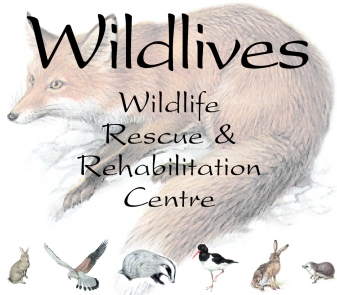This image, featuring a white background, appears to be a logo or promotional graphic for a group called "Wildlives Wildlife Rescue and Rehabilitation Center." Dominating the center is a large fox, possibly a red fox, positioned facing left. The fox is depicted with a partial white translucency, lending it a subtle, almost ethereal quality that integrates it into the background yet distinguishes it in color. 

Below the fox, a series of smaller, detailed illustrations of various animals are aligned along the bottom. Starting from the left, there is a gray rabbit sitting upright. Next to it is a bird of prey, likely an eagle or a hawk, characterized by its dark, two-toned wings and large white tail feathers tipped in black. To the right of this bird is a badger, or possibly a honey badger, shown on all fours with its snout facing downward. Further along is a black-and-white bird distinguished by a long, narrow, orange beak, standing with one leg raised. Following this bird is a brown hare with long, upright ears, its body facing right while its head is turned left, appearing alert. Finally, there is a small rodent, perhaps a shrew or mole, with gray coloring and white markings around its face and chest.

The text "Wildlives" is prominently displayed over the fox, with "Wildlife Rescue and Rehabilitation Center" written below in black font, providing a clear and descriptive naming to the image's purpose.